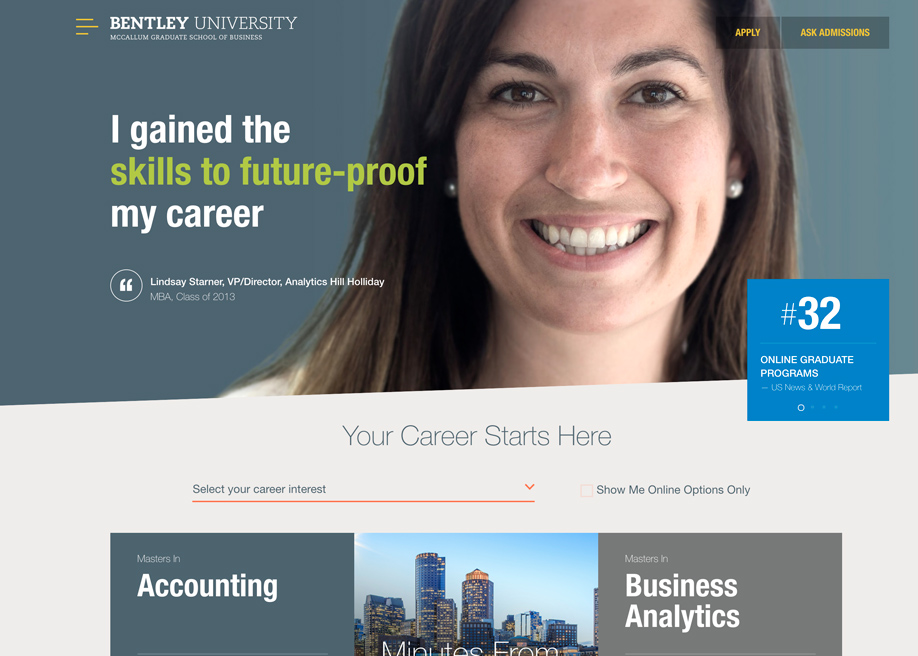The image showcases the landing page for Bentley University's McCallum Graduate School of Business. At the forefront, a female model is smiling, adding a warm, engaging element to the page that draws visitors' attention and humanizes the digital environment. Prominently displayed is a box highlighting Bentley's impressive #32 ranking in online graduate programs. 

Further down the page, notable fields of study such as "Big Texan Accounting" and "Masters in Business Analytics" are mentioned, emphasizing their popularity and relevance in today's academic landscape. 

The page is text-heavy, featuring the Bentley University logo and "McCallum Graduate School of Business." Key call-to-action buttons like "Apply" and "Ask Admissions" are strategically placed to facilitate user navigation. Highlighting Bentley's impact on careers, a quote from Lindsay Starner, a 2013 MBA graduate and current VP and Director of Analytics at Hill Holliday, reads, "I gained the skills to future-proof my career."

At the bottom, the page encourages prospective students with the phrase "Your career starts here," alongside a drop-down menu to select a specific career of interest, likely leading to more detailed information on relevant curricula and programs.